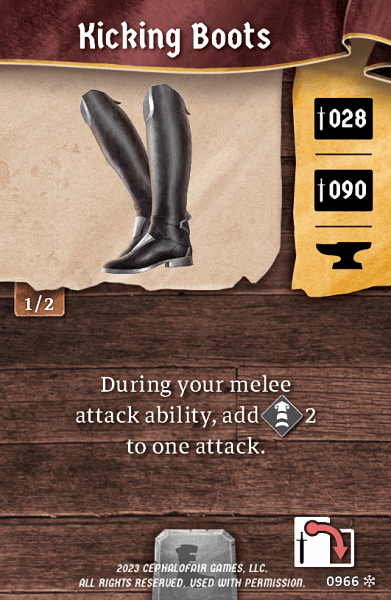In this image of a video game item interface, the focus is on an item tab displaying a pair of boots, specifically named "Ticking Boot." At the top of the interface, there is an ornate maroon banner with the item name "Ticking Boot" prominently displayed in the center. Below the banner, a detailed image of black boots is featured, indicating the item's appearance in the game.

To the right of the boots, there is a section divided into three parts with a yellow background. Each part contains different information related to the item's stats. The first part has a black box with a small white sword icon, followed by the number "028." There’s a vertical line separating this from the next part, which similarly has a black box with a white sword icon, followed by the number "090." The third part consists of a black anvil icon.

Below this section is a wooden board-like area where the item’s descriptive text and capabilities are displayed in white letters. It reads: "Doin Yimili Attack Ability. Add two armor. Add two to one attack," accompanied by a gray diamond icon featuring white armor, indicating a boost in both defense and offensive capabilities.

At the bottom of the interface is a small gray button, along with two white boxes connected by an arrow that points to a black sword in the middle, suggesting some form of interaction or enhancement option.